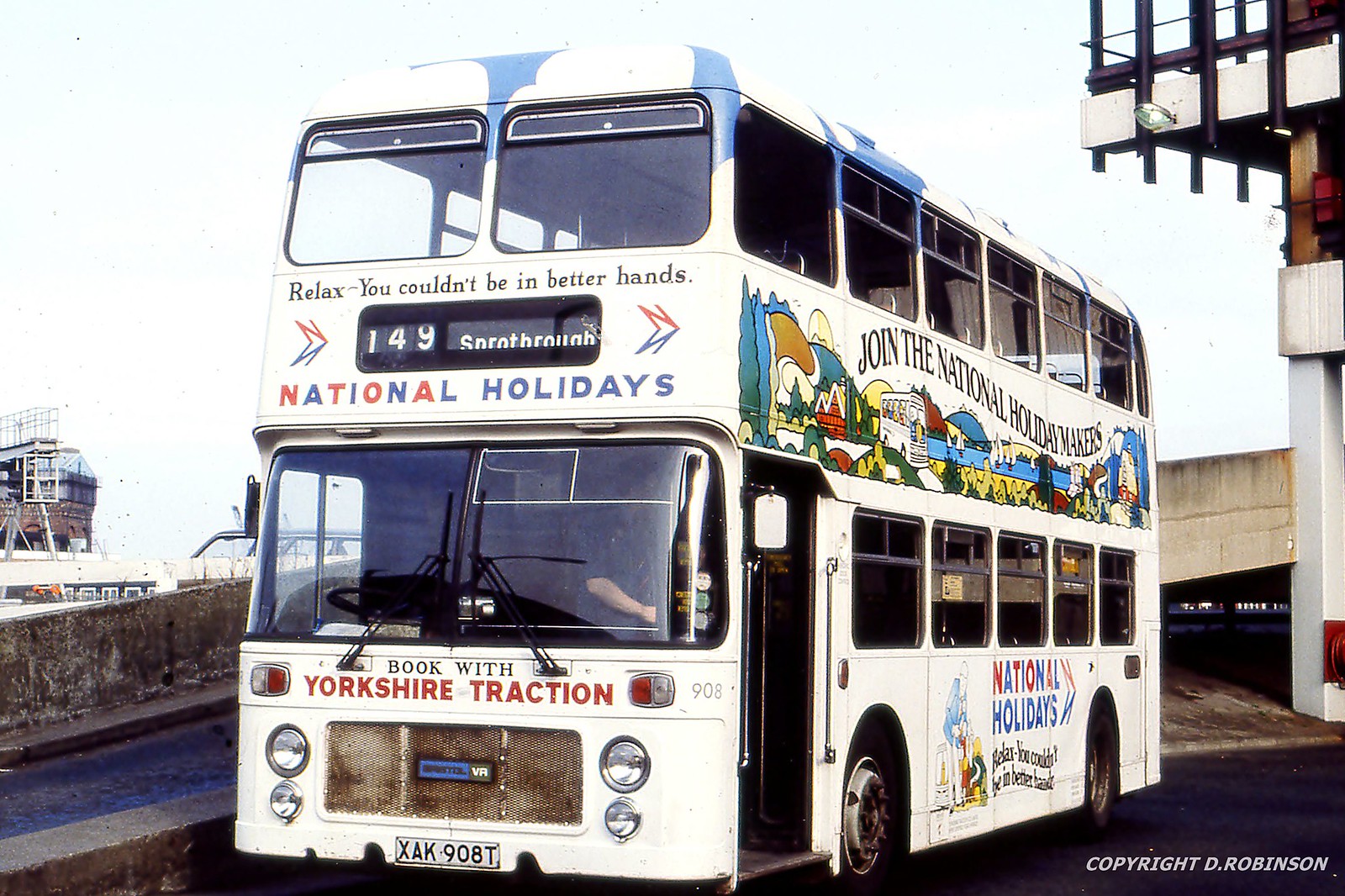The photograph captures an older, white double-decker bus parked in a dingy urban setting, possibly adjacent to a concrete on-ramp or parking garage. The bus is adorned with various texts and graphics: the top of the front reads "Relax, You Couldn't Be In Better Hands" in black font, followed by "National Holidays" underneath. Near the bus driver's window, there's a red-lettered message, "Book with Yorkshire Traction." The side of the bus features the phrase "Join the National Holiday Makers," accompanied by a mural between the upper and lower levels, with some graphics possibly including clouds. The license plate reads XAK 908T. Some of the bus windows appear to be open or missing. A person, potentially the driver, seems poised to step out of the bus. The backdrop includes a bridge and a building, indicating daytime. The photograph credits D. Robinson for the capture.